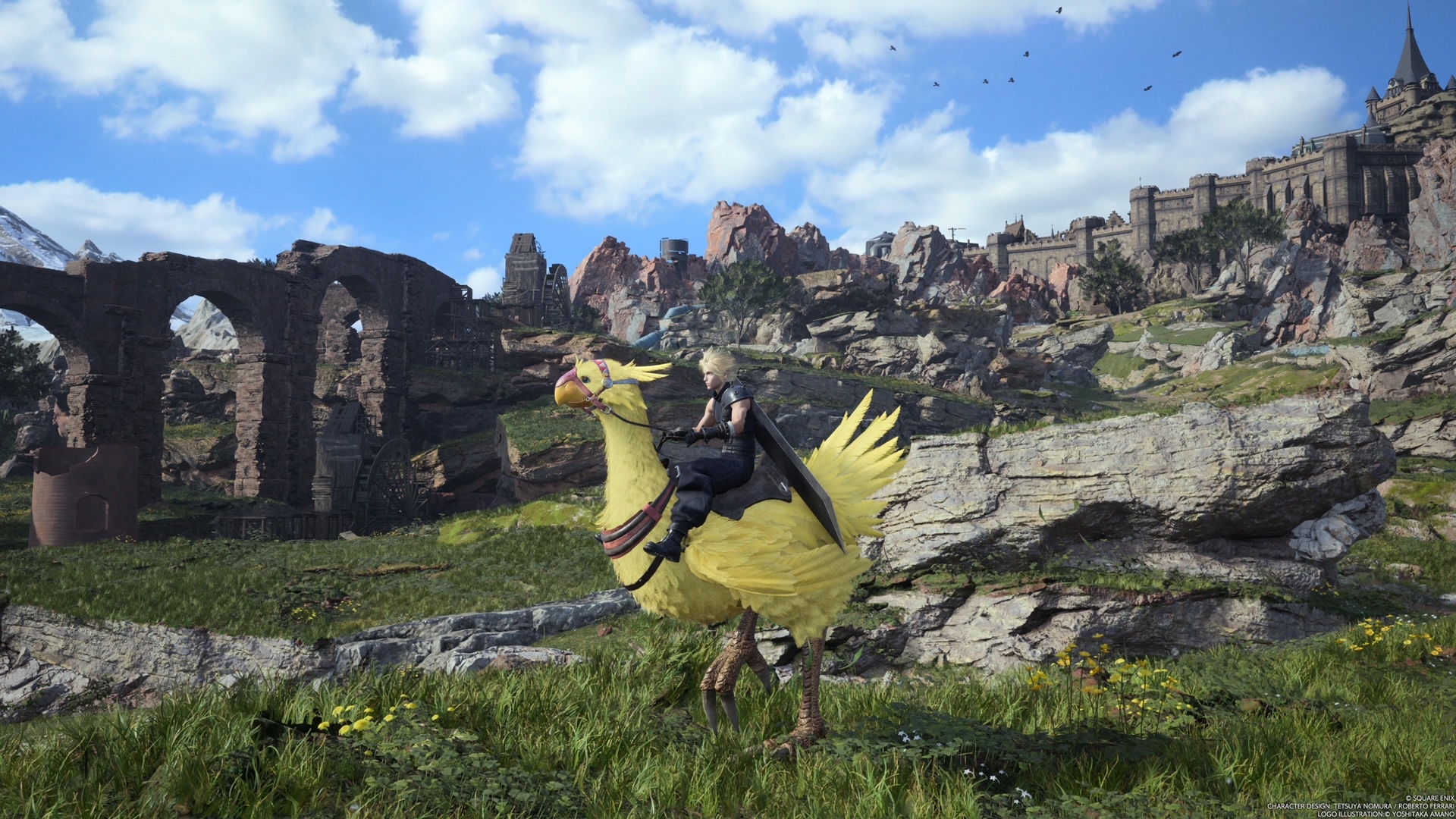In this detailed scene from a video game, a character—a girl with short blonde hair, dressed in a uniform—rides a large, yellow bird similar to an emu, or a huge duck, with distinctive large feet. The setting is an outdoor environment under a clear blue sky adorned with a few white clouds and birds flying. The landscape features lush grass, scattered dandelions, and lots of rocks amidst what appears to be ancient Roman ruins. These ruins include stone buildings with archways and an aqueduct. In the distance, an imposing castle stands against the sky, contributing to the sense of antiquity and grandeur. The entire scene feels meticulously crafted, resembling an artistic depiction or animation, reminiscent of a setting one might find in a Final Fantasy game.